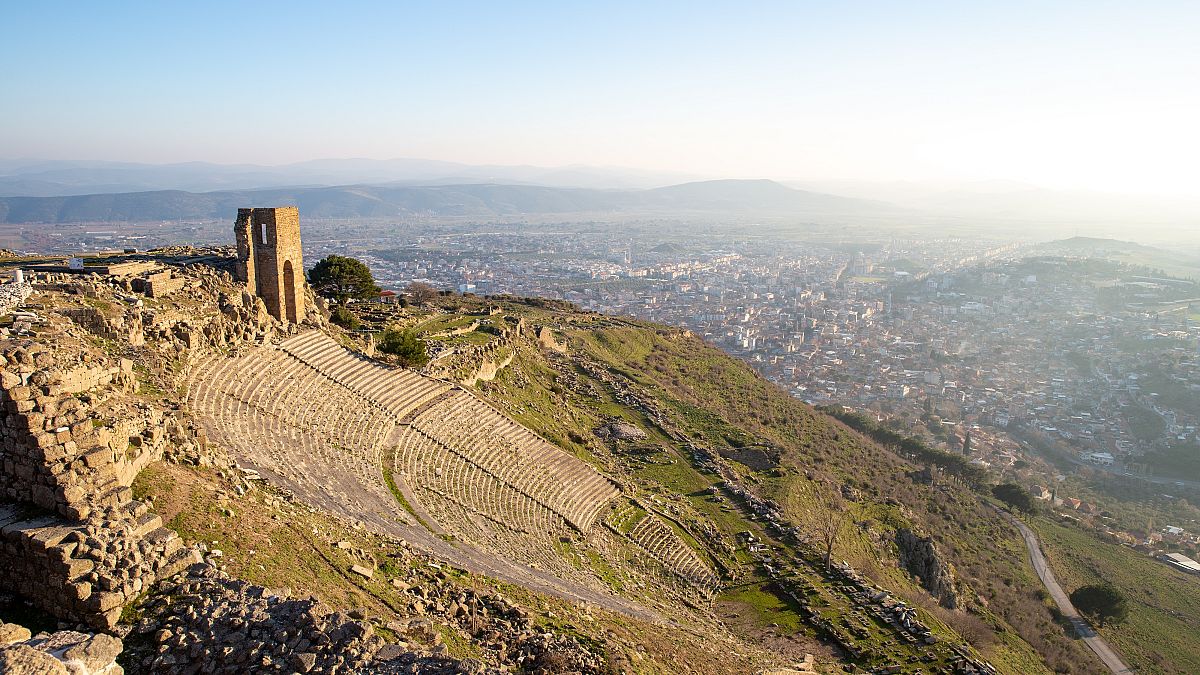The image captures a vivid daytime aerial view of an ancient amphitheater situated atop a hill, likely taken from a drone. The amphitheater, built with brown stones, exhibits three distinct seating sections cascading down the hillside, with tiers closest to the stage, a middle section, and the highest tier at the top of the hill. To the left of the amphitheater, there's a structured stone pillar featuring an entryway. The foreground is characterized by a mix of green terrain and some sporadic brown dirt patches. A roadway meanders through the bottom right area of the image. Surrounding the amphitheater, there's a modern cityscape nestled in a valley with numerous homes clustered together, framed by large hills and distant blue mountains. The bright blue sky and natural daylight amplify the clear quality of the scene, accentuating the stark contrast between the ancient ruins and the urban environment below.